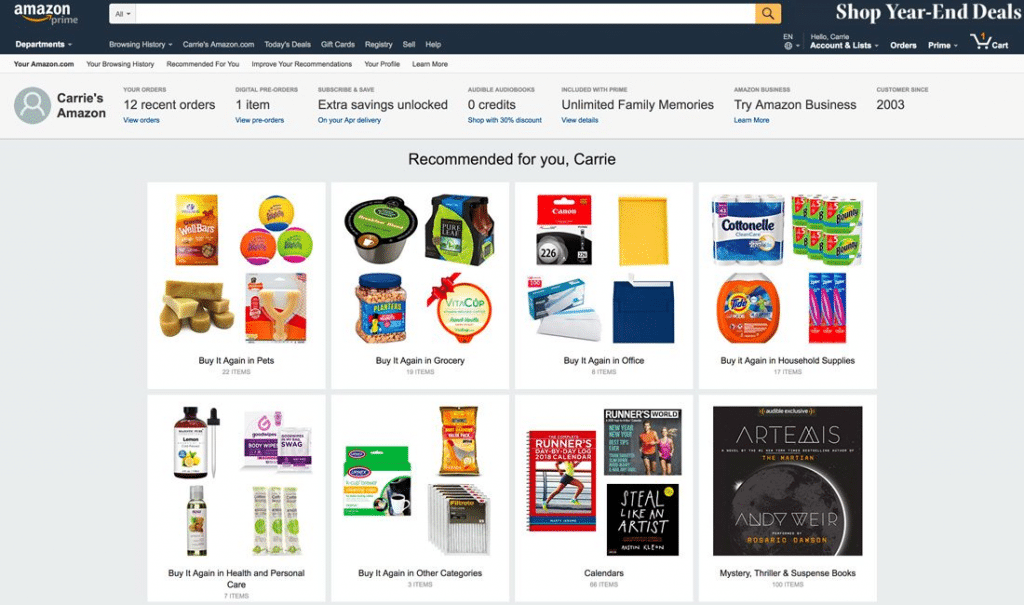This image showcases the Amazon shopping app, specifically an Amazon Prime account. At the top right corner, the "Amazon Prime" label is prominently displayed, indicating active membership. Directly below the Prime label, the account is named "Carey’s Amazon."

The interface at the top includes various tabs and sections: "12 Recent Orders," "One Item," "Extra Savings," "Loss," "Zero Credits," "Unlimited Family Memories," "Try Amazon Business," and "2003." These options offer a glimpse into the user's recent activity and available resources.

Further down, the section titled "Recommended for you, Claire" features an array of personalized recommendations. The first category displayed is "Buy It Again in Pets," which includes 22 items. Following this, there are recommendations for "Buy It Again in Grocery," with 19 items, and "Buy It Again in Office," with 6 items. The "Buy It Again in Household Supplies" section showcases 17 items.

The next row begins with "Buy It Again in Health and Personal Care," featuring 7 items, and continues with additional categories such as "Calendars" and "Mystery, Thrillers, and Suspense Books." This visually rich interface highlights Amazon's tailored suggestions based on the user’s past purchases and browsing history.